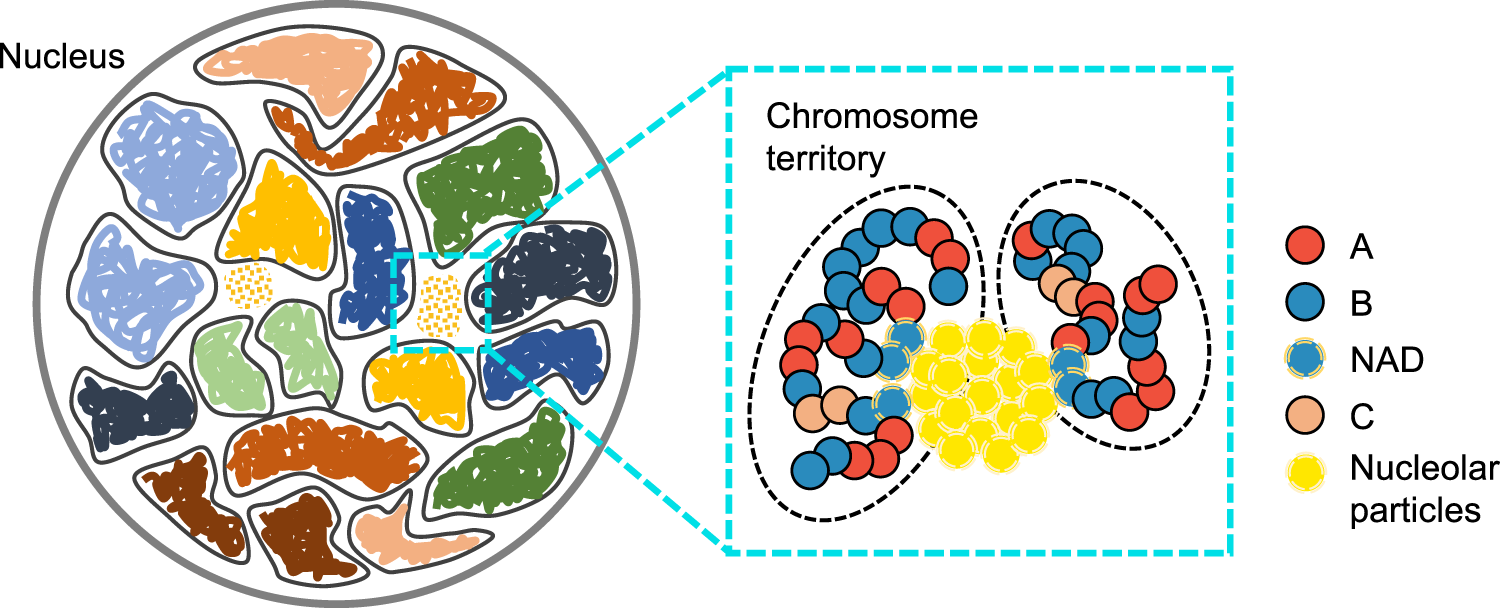The image is a detailed infographic depicting the structural components of a cell, with a focus on the nucleus and its various parts. The central feature of the infographic is a diagram of a cell's nucleus, highlighted by its key components: the nucleus itself and the chromosome territory. The chromosome territory is distinguished by a bright teal or turquoise color and is prominently labeled.

To the right of the nucleus diagram, there is a color-coded key that explains the significance of the colors and shapes used within the image. According to the key, red indicates 'A', blue denotes 'B', a specific splotchy shape represents 'NAD', tan stands for 'C', and yellow highlights nuclear particles. 

In addition, the infographic includes a magnified section of the chromosome territory, marked by a square made of dotted lines, which provides an enlarged view of this specific area. This section reveals oval shapes containing chains of colored circles, further illustrating the intricate details within the chromosome territory.

Overall, the infographic, although cartoony in its style, serves to visually represent the important regions and components within the nucleus, using a distinct and accessible color and shape coding system.